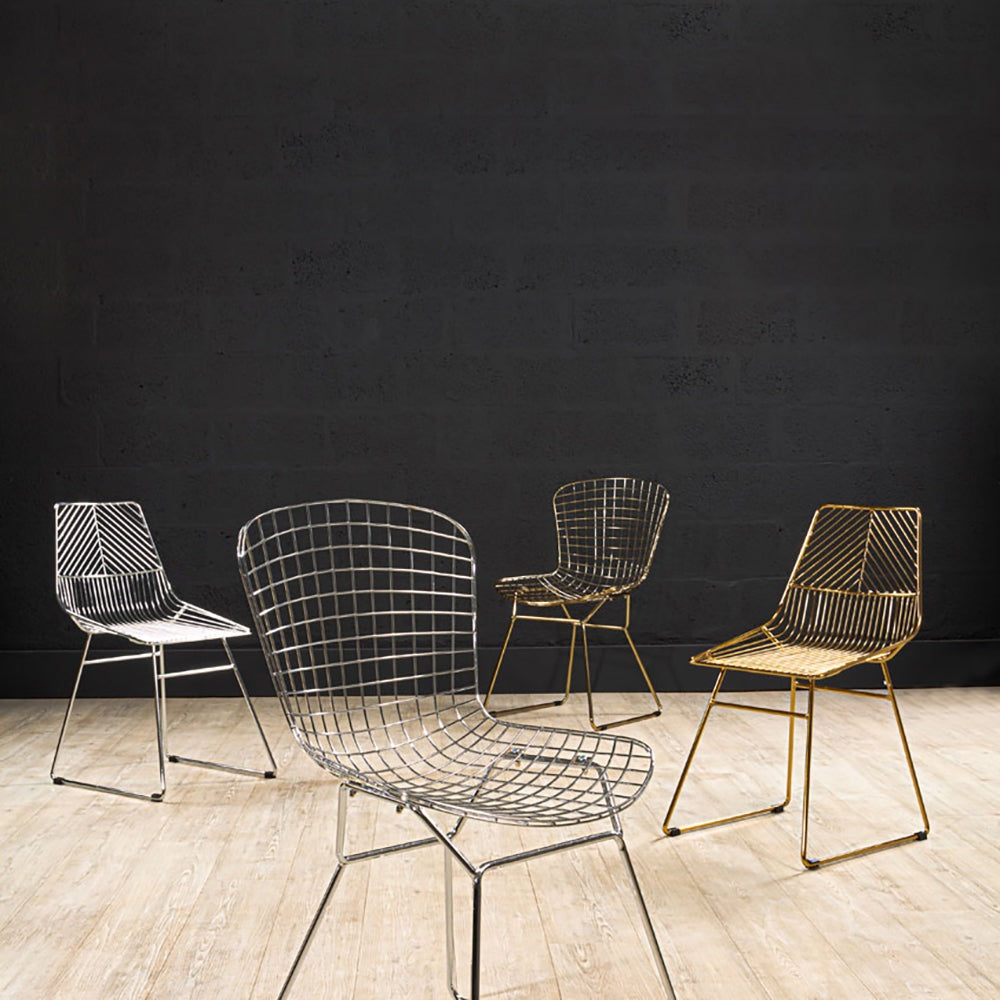The photograph depicts an interior space, possibly a warehouse or an art design studio, characterized by its distinctive black cinder block walls and light-toned hardwood floors with a subtle pinkish, creamy hue. In the room stand four metallic chairs, each pair sharing the same design but differing in finish—one pair is gold, the other stainless steel. On the left, the two chairs feature a flat back and sides, with a shovel-like seat. Opposite them, the other pair has a more intricate design, with a rounded back and seat formed by a grid of squares. The arrangement and design of the chairs, coupled with the unique backdrop, create a striking and modern aesthetic.